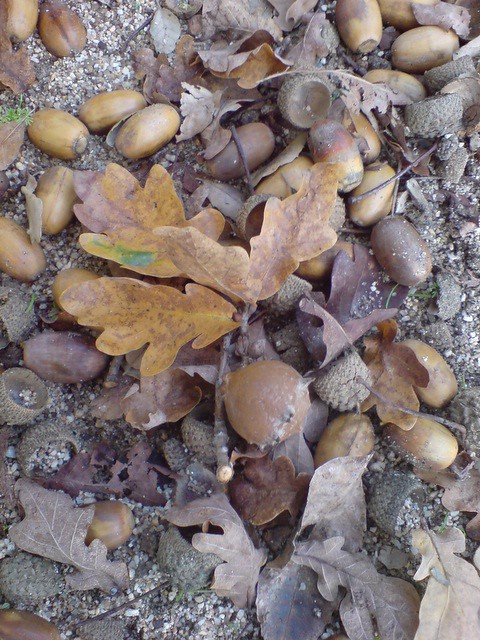The photograph captures a diverse and detailed ground scene featuring a mound of leaves, tree remnants, and acorns scattered about. Central to the image is a branch adorned with a mix of brown and slightly green leaves. Various darker leaves are dispersed towards the bottom. Numerous small acorns, some with their cups and others without, are prominently visible, particularly towards the upper section. Light brown and dark brown acorns coexist, some appearing broken or partially eaten, adding to the texture. Intermixed with the leaves are fragments that resemble parts of pine cones or acorn shells. The base of this natural composition is a gravelly surface, evident through small patches of visible dirt and gravel. The array of oak leaves, varying from yellowish-brown to dark brown, adds to the autumnal aesthetic of the photograph.